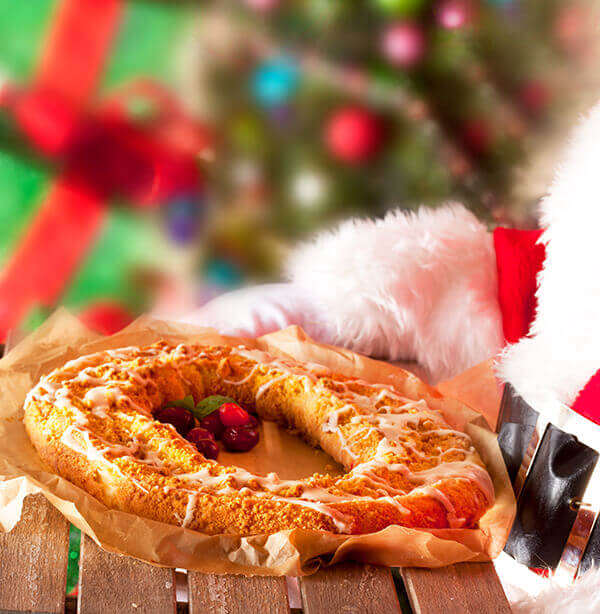This image is a close-up of a festive scene centered around a delectable pastry. The pastry is circular in shape, made of brown bread, and lavishly drizzled with white cream. In the middle, dark round berries and green leaves add a natural, colorful touch. The pastry rests on a thin brown paper atop a rustic wooden tray composed of several brown slats.

A Christmas tree adorned with ornaments and a green present wrapped in a red ribbon are slightly out of focus in the blurred background, adding to the holiday ambiance. To the right, a figure dressed in a Santa suit is visible from the waist down, characterized by a red outfit trimmed with plush white fur, a wide white belt with black accents, and white gloves. The Santa figure is holding the tray, presenting the pastry as a festive offering, while a hint of white and red—perhaps part of the Santa costume—can be seen in the background, contributing to the overall Christmas theme.